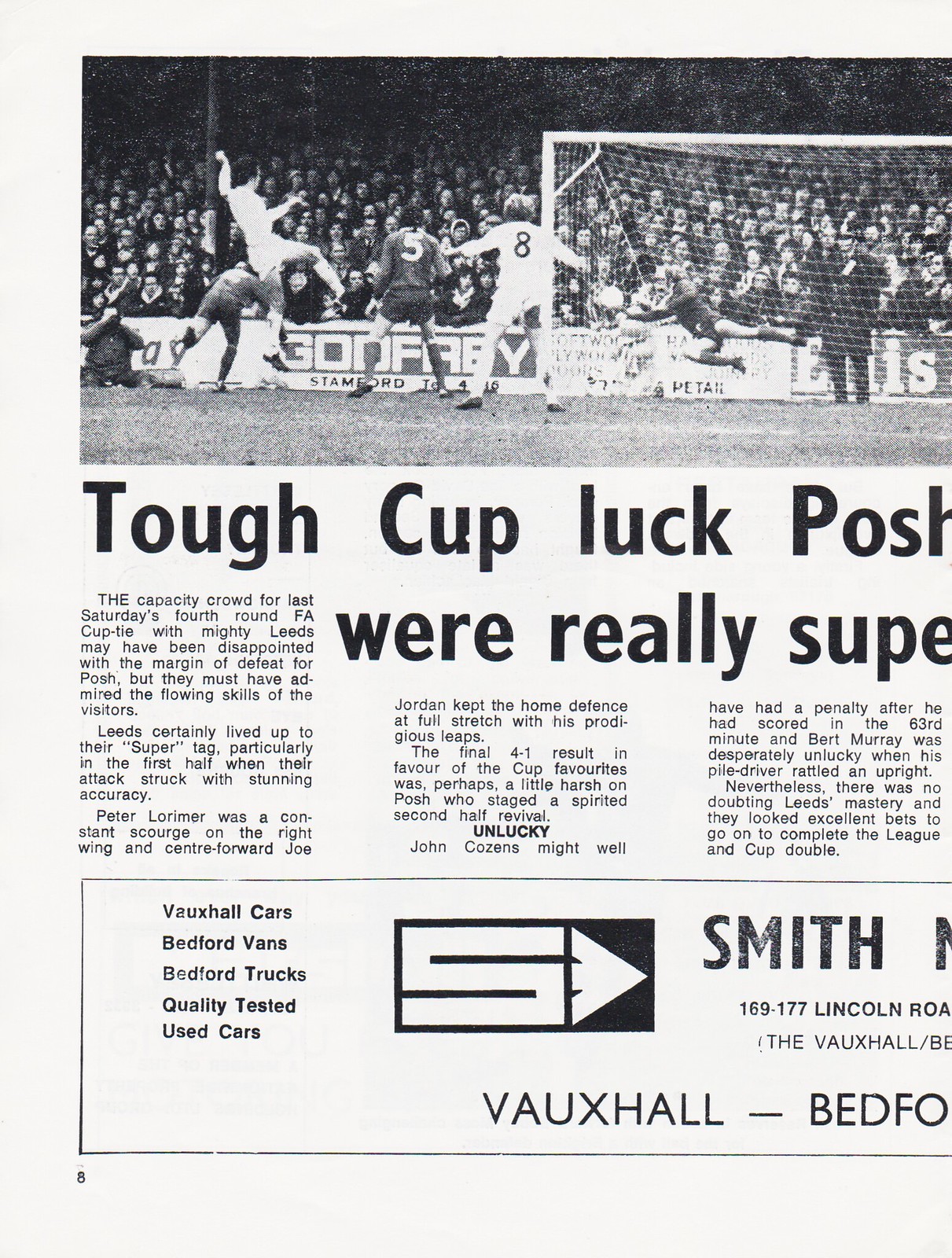The image is a photocopy of an old newspaper cutout featuring a dynamic soccer match scene. The photograph captures the intense moment as a goalie leaps mid-air to intercept the ball, while players from both teams energetically contest for possession. In the background, spectators packed in the stands keenly watch the action unfold. The partially visible title of the article reads, "Tough Cup Luck Posh" or something similar like "We're Really Super." The accompanying article discusses a fourth-round FA Cup tie between Leeds and another team, referred to as "posh." The crowd witnessed Leeds demonstrate their top-tier skills, especially in the first half when players like Peter Lorimer and Joe Jordan dominated the field, ending the match with a 4-1 victory over posh, who mounted a spirited second-half comeback. At the bottom of the page, there is a detailed advertisement for Vauxhall Cars, Bedford Vans, Bedford Trucks, and quality-tested used cars available on 169-177 Lincoln Road, Fox Hall.